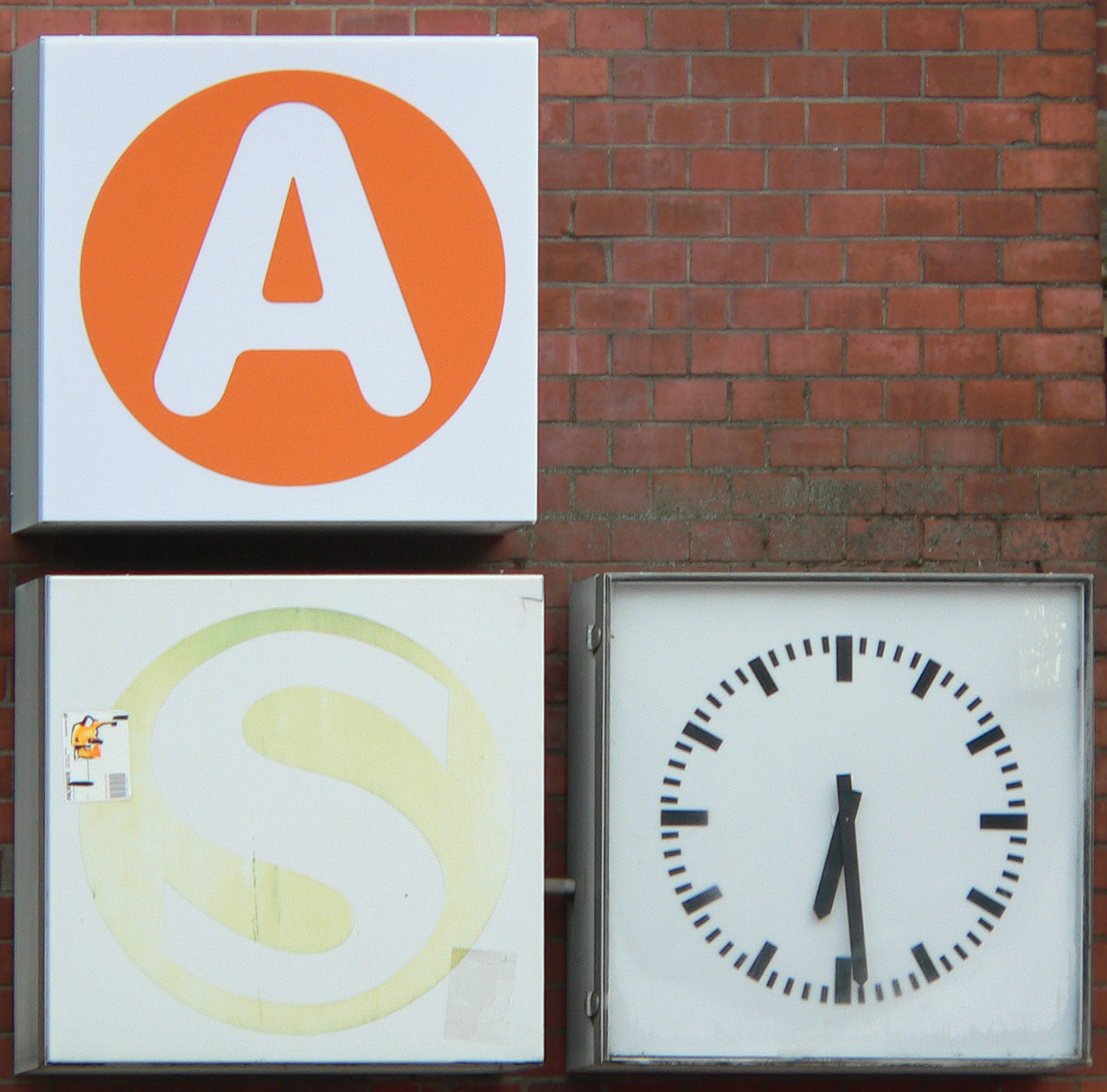This image depicts a brick wall adorned with four distinct, white, square objects. 

1. In the top left corner sits a white box featuring a large, white 'A' cut out from an orange circular insert.
2. Directly below, in the bottom left corner, there's a black box with a similar white 'S' cut out from a yellow circular insert. This box appears to have a piece of tape affixed to its surface, displaying what looks like an orange and black, potentially barcoded detail along with other indistinct black markings.
3. In the bottom right corner, there's a square clock encased within a hinged, square metal frame, likely made of plastic or glass. The clock face is white, adorned with black tick marks instead of numbers, and has black hour and minute hands. 

Each object stands out against the brick background, presenting a blend of geometric and color contrasts.